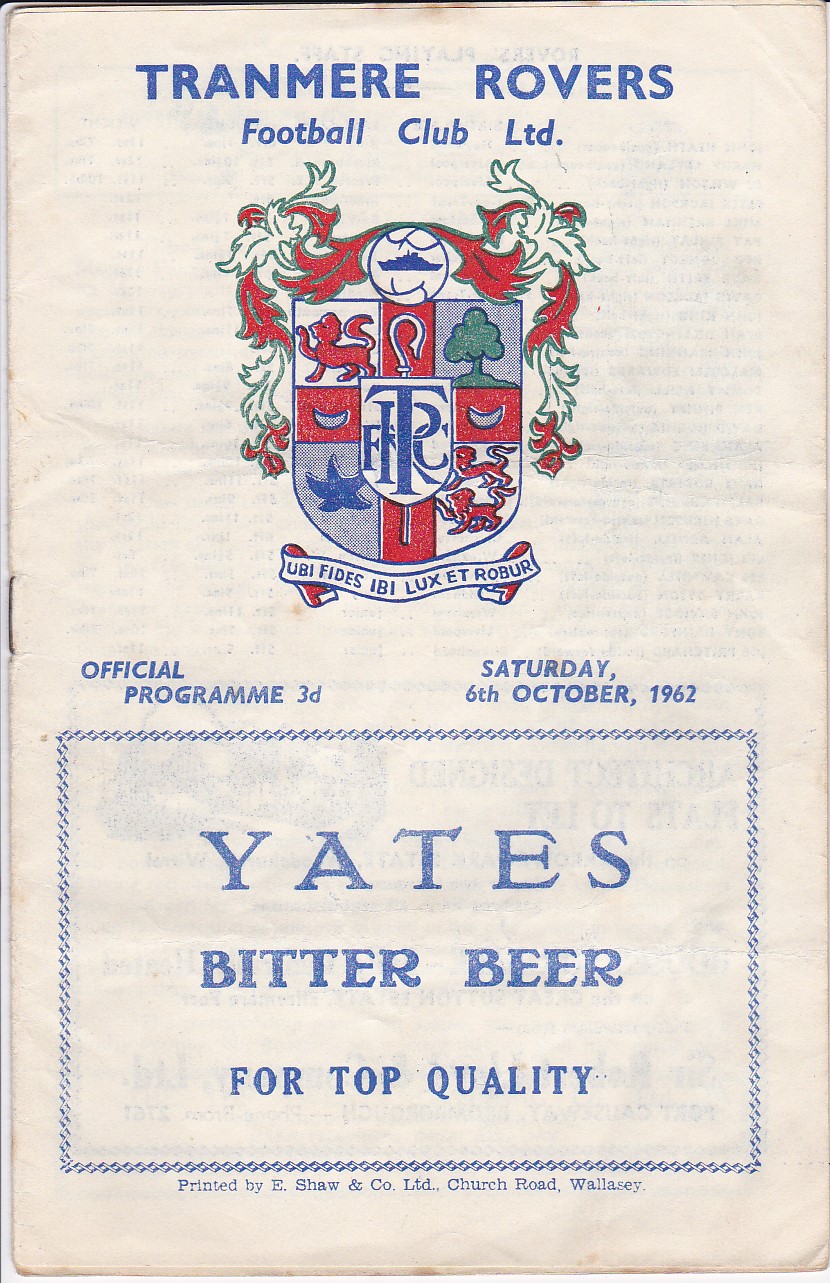The image depicts the cover of an official program for the Tranmere Rovers Football Club Limited, dated Saturday, October 6, 1962. The program, which measures approximately 3 by 5 inches, is stapled with a single staple in the middle for binding. At the top of the cream-colored cover, "TRANMERE ROVERS FOOTBALL CLUB LIMITED" is printed in blue letters, accompanied by an elaborate club emblem featuring a shield with red, blue, and green colors, and a ribbon beneath it bearing the motto "UB FIDES EB LUX ET ROVER." Below the emblem, "OFFICIAL PROGRAM 3D" is printed, with "3D" denoting its price. Further down, encased in a blue rope-design border, is an advertisement for "YATES BITTER BEER," promoting its top quality. At the very bottom, the program notes it was printed by Eshaw and Company Limited, located on Church Road, Wallasey, UK.